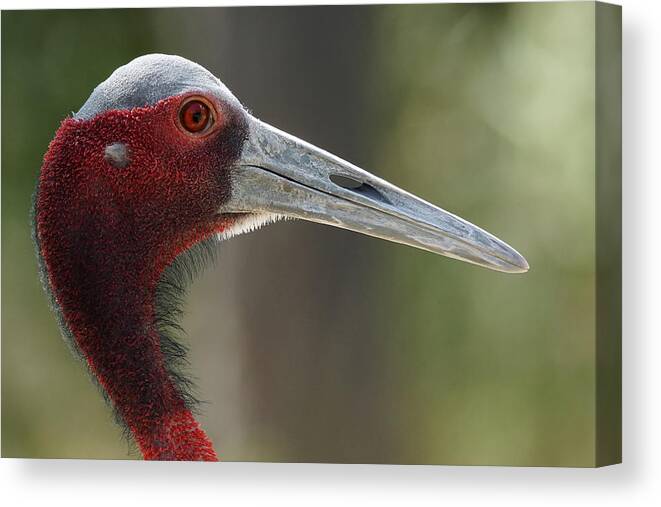The image features a close-up view of a bird's head and upper neck, facing to the right. The backdrop appears bright and blurred, likely indicating an outdoor setting with hints of greenery, although another interpretation suggests a white background with a canvas shadow. The bird's head is notably small with a crown of gray feathers. Its skin around the neck and eyes is a striking red, with a bumpy, less-feathery texture. Red eyes with black pupils bring a vivid contrast to the overall appearance. The bird's beak is elongated and gray, featuring a pronounced nostril near the middle. Black, hair-like feathers are visible under the cheeks, extending into the red skin area and adding to the detailed textures depicted.